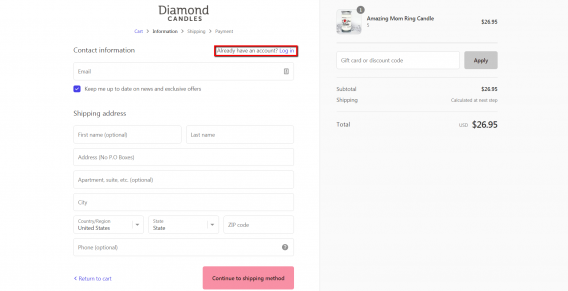The image displays a light-colored rectangular layout divided into two sections. On the left section, near the top, there is small, light gray text on a white background reading "Diamond Candles," with "Diamond" in a larger font than "Candles." Below this are two lines of text, the second of which says "Contact Information." Adjacent to this is a red-outlined box labeled "Login." 

Further down, there is a box likely intended for entering an email address. Below this, there is a blue box with a check mark next to text stating "Keep me up to date on offers," or something similar. Following this is a section to input a shipping address. At the bottom of this section, there is a pink box that says "Continue to Shipping," though the exact wording is somewhat unclear.

The right section features a product labeled "Amazing Mom Ring Candle," accompanied by a small image of the item and a price tag of $24.95. There is an area for applying a discount code, followed by details showing the subtotal, shipping cost, and total amount due. The rest of this vertical rectangle on the right side is shaded in gray.